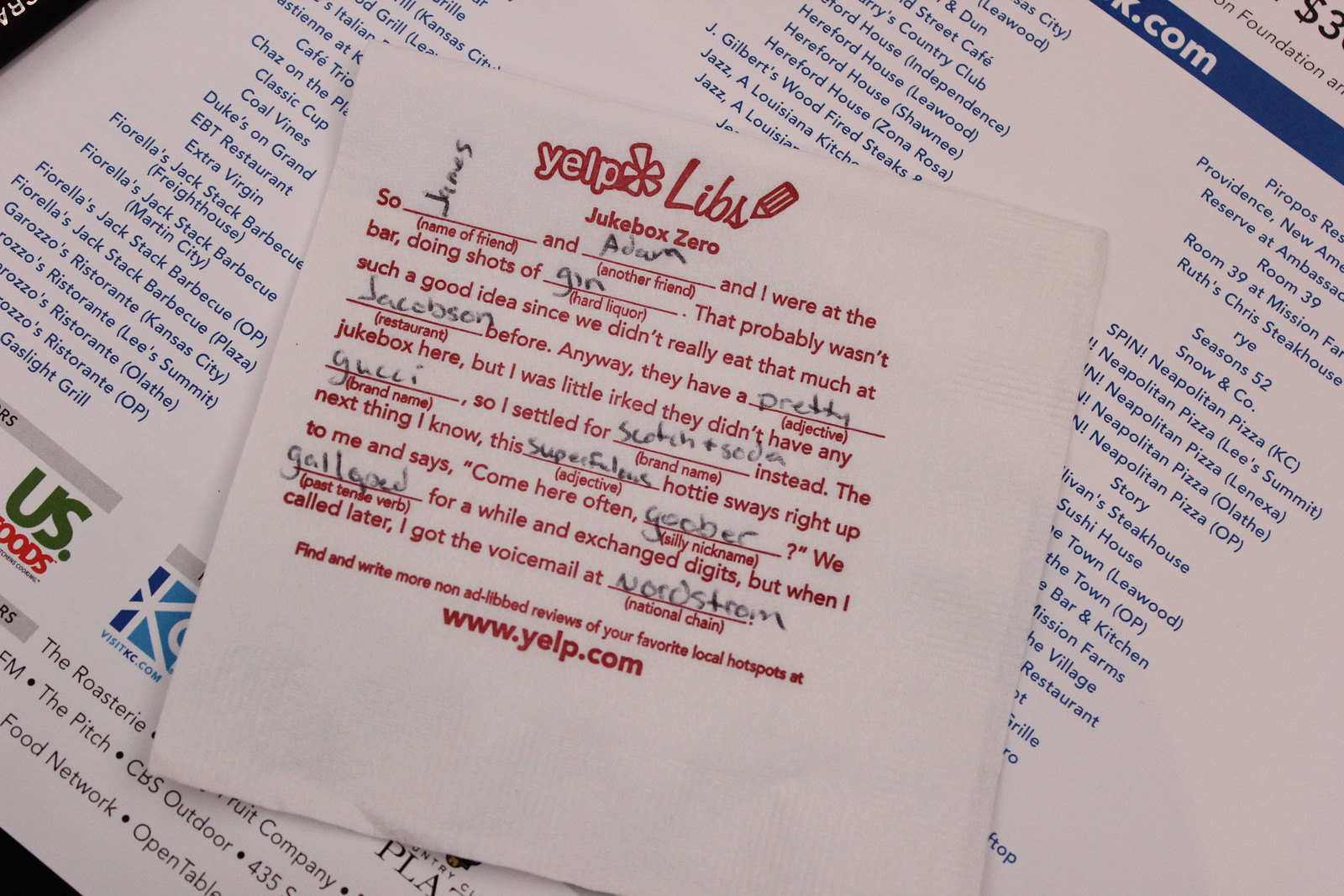This photograph captures a unique promotional napkin from Yelp laid atop what appears to be a restaurant menu background. The square, white napkin features red lettering, starting with the Yelp logo followed by "Yelp Libs" in cursive next to a pencil emoji, and then "Jukebox Zero." Below this, in a playful Mad Libs format, is a story inviting people to fill in the blanks: "So [Name of a friend] and [Another friend] and I were at the bar doing shots of [Name of liquor]. That probably wasn't such a good idea since we didn’t really eat that much at [Name of a restaurant] before." The placeholders are filled with handwritten entries in black ink, such as "James," "Adam," and "Gin." The story continues with personalized adjectives and band names, revealing an engaging and humorous narrative. At the bottom of the napkin is a call to action, directing users to "Find and write more non-ad-lib reviews of your favorite local hotspots at www.yelp.com." The restaurant menu beneath the napkin has a white background with blue text, listing several menu items and featuring a blue bar with a barely visible website URL at the bottom.